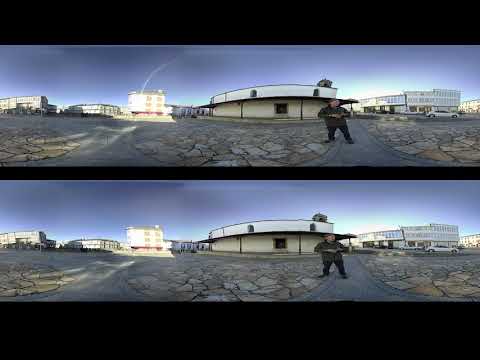The image depicts a cold, gray-blue day within an outdoor plaza, represented twice in a layered, panoramic format separated by thin black bars. Dominating the foreground is a man dressed in black, standing on an intricate pathway composed of gray, blue, brown, and white cobblestones. He's positioned slightly to the right of the center, with his hands in front of his chest, looking off to the side. The scene features a semi-circular white building behind him, marked by a single dark opening, and adorned with a covered black overhang. This building is overlooked by a brighter white or silver-gray vehicle parked in front of it. On the right, additional white multi-story buildings stand clustered, and on the left, more multi-story structures, one shimmering under direct sunlight. Both iterations of the image highlight subtle variations, such as differing lighting on the buildings and slight changes in the man's pose against the backdrop of a cloudy, placid sky.